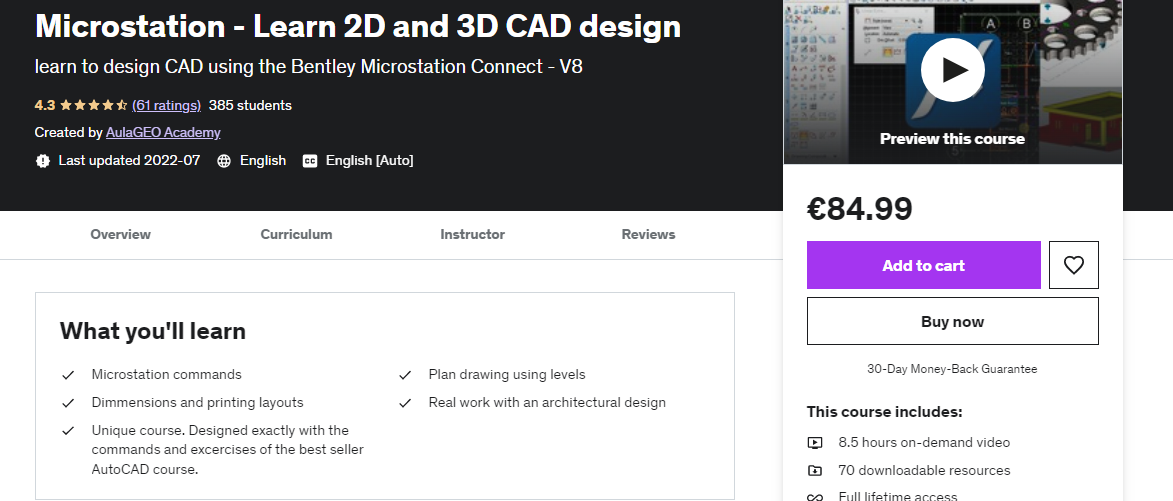**Detailed Caption for the Screenshot from a Webpage:**

The image is a screenshot from a webpage that features a dark black rectangle as the primary background. On the left-hand side of this black rectangle, bold white text reads "MicroStation - Learn 2D and 3D CAD for CAD Design". Below this, in regular white text, it states, "Learn to Design CAD using the Bentley MicroStation Connect Edition". The description specifies that the course is for the "MicroStation V8" version. The course rating is displayed prominently, showing "4.3 out of 5 stars" with the number "4.3" and the stars in gold. Following this, in violet text and parentheses, it notes that there are "61 ratings".

Further down, in white text, it is indicated that the course has "385 students" enrolled. Below this figure, in white text, it says "Created By" followed by the creator’s name, "Auto Ola GEO Academy" in violet and underlined.

Continuing down, there is a white star-like circle containing a black exclamation mark, adjacent to white text that reads, "Last Updated 2022-07", signifying the course was last updated in July 2022. Next to this is an icon of a globe with longitudinal and latitudinal bands, accompanied by the text "English". Additionally, there is a closed captioning symbol, a white square with black lowercase "c"s inside, next to the word "English" in white, followed by "Auto" in brackets.

On the right-hand side of the black rectangle, a segment of a video is visible with the overlay text "Preview this course" in bold white. The preview shows multiple open windows with a gray background featuring a gear icon, and in the center is a white circle with a black right-pointing play button. Below that, it mentions the cost of the course as "84.99 Euros". A purple-violet rectangle with bold white text says "Add to Cart". Beneath this, a black-bordered square contains a black heart symbol, and a similarly bordered rectangle below lists in bold black text "Buy Now". Below this, in gray, it provides information about a "30-day money-back guarantee". Further down in bold black text, it reads "This course includes...". The inclusion details state "8.5 hours on-demand video" with an overturned black triangle, "70 downloadable resources" with a black folder and down arrow icon, and "full lifetime access" symbolized by an infinity symbol.

Under the black rectangle, various tabs in dark gray or black are displayed, labeled "Overview", "Curriculum", "Instructor", and "Reviews". Beneath this section, there is a rectangle outlined in thin gray, with bold black text that reads "What You'll Learn". Following this, there are several check marks followed by text detailing course content: "MicroStation Commands, Dimensions, and Printing Layouts", "Unique Course, Design Exactly What the Command and Exercises of the Best-Seller AutoCAD Course", and "Plan Drawing Using Levels". The subsequent repetitive entries mistakenly list "Drawing Using Levels" three more times. Finally, the list concludes with a point stating "Real Work with an Architectural Design".